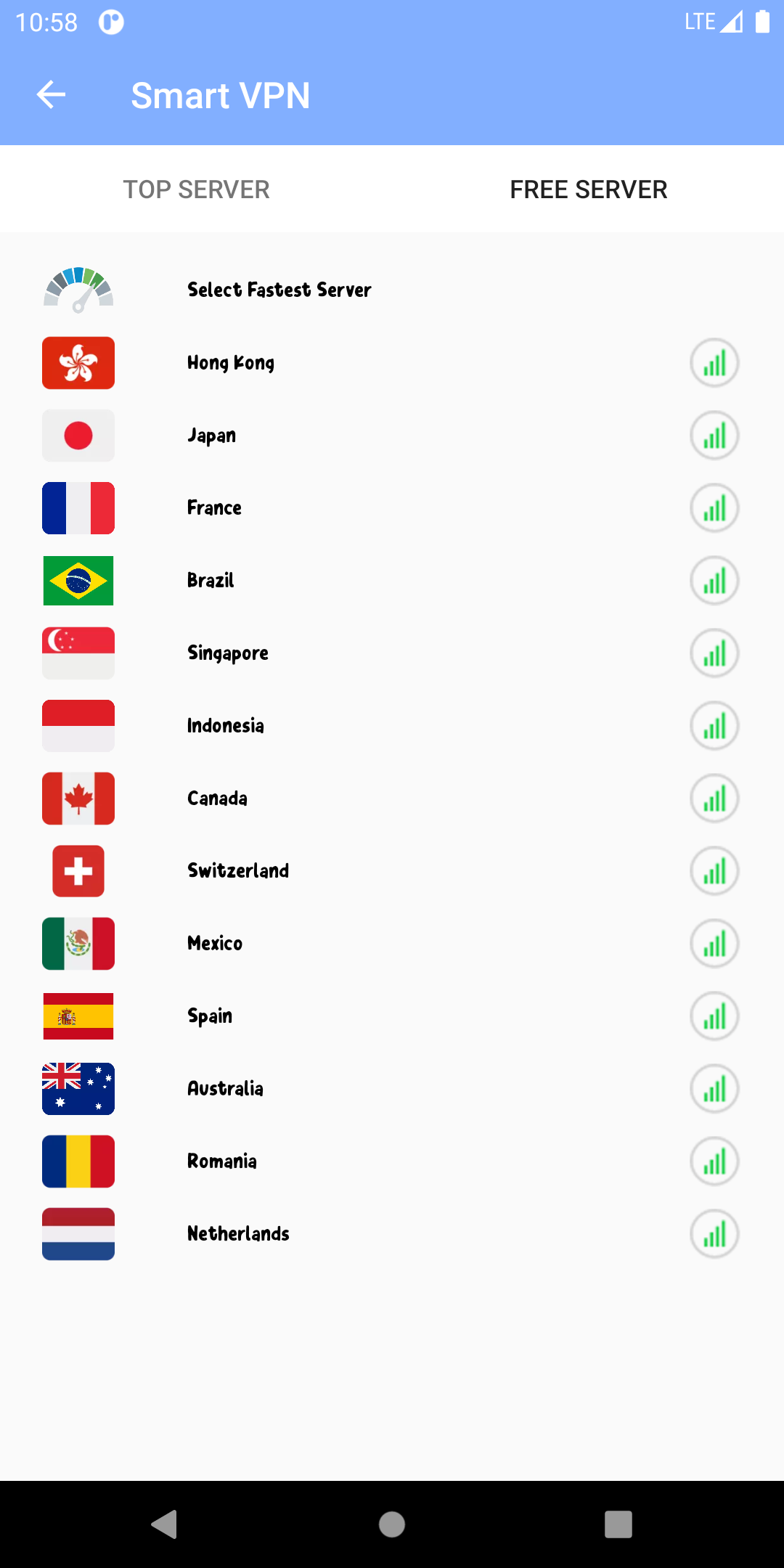A detailed screenshot captured on a smartphone in vertical orientation displays a phone interface at 9:58 AM. The top toolbar includes essential phone status icons: the time on the far left, followed by a circular indicator with the letter 'R,' and on the right side, connectivity indicators like LTE and a partially filled triangle, alongside the battery icon. Below the toolbar, a blue banner reads "Smart VPN" with a left-pointing arrow, indicating navigation.

The main interface features two tabs: "Top Server" and "Free Server," with "Free Server" bolded, indicating the active tab. Under this section, a vertical list of server options is displayed, each entry comprising a country flag on the left, the country's name in bold on the right, and on the far right, a gray circle displaying ascending vertical lines in green, likely signifying data availability or signal strength.

The first option, "Select Fastest Server," includes an icon resembling a speedometer with varying shades of gray, blue, and green, depicting a dial pointing to dark green—suggesting it identifies the fastest available server. Following this, the list of countries available for VPN selection includes flags and names of Hong Kong, Japan, France, Brazil, Singapore, Indonesia, Canada, Switzerland, Mexico, Spain, Australia, Romania, and the Netherlands, each equipped with similar indicators for data or signal strength.